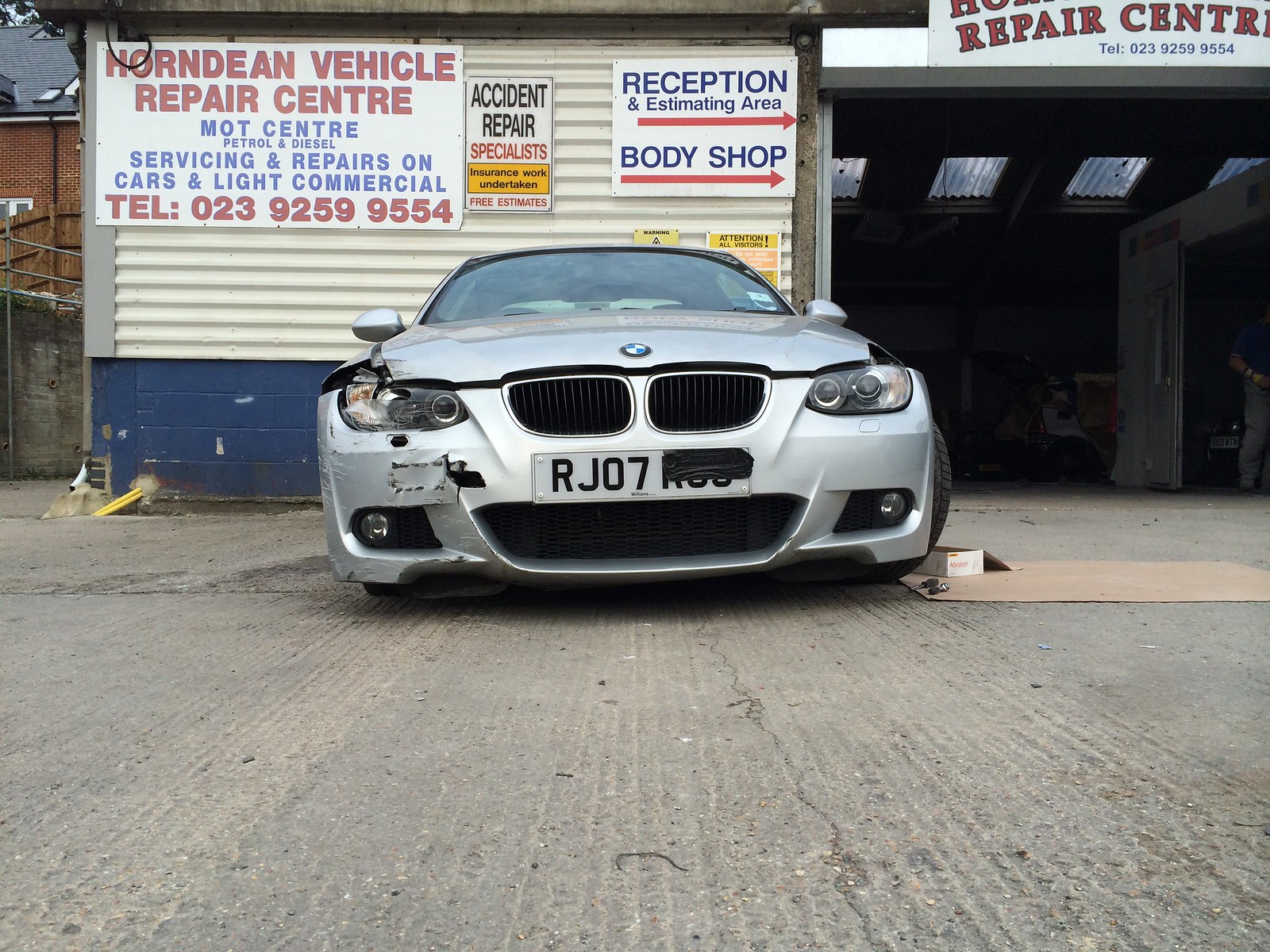The image is an outdoor scene taken at a low angle, level with the front of a gray BMW that appears to be parked on a concrete or paved surface in front of a repair garage. The BMW has noticeable front-right damage, particularly to the bumper, headlight, and hood, suggesting it was recently in a crash. The license plate reads "RJ07," but the last three characters are obscured.

Behind the car is a building with a cinder block base and a metal upper section, painted blue and silver. Prominent signage on the building reads "Horn Dean Vehicle Repair Center." Additional signs provide details such as "Servicing and repairs on cars and light commercial," "Mod Center, Petrol and Diesel," and the telephone number "023-9259-9554." Smaller signs indicate services like "Accident Repair Specialists," "Insurance Work Undertaken," "Free Estimates," and direct to "Reception Estimating Area" and "Body Shop." The open garage bay reveals more of the repair shop's interior, emphasizing that the shot was taken during the day.